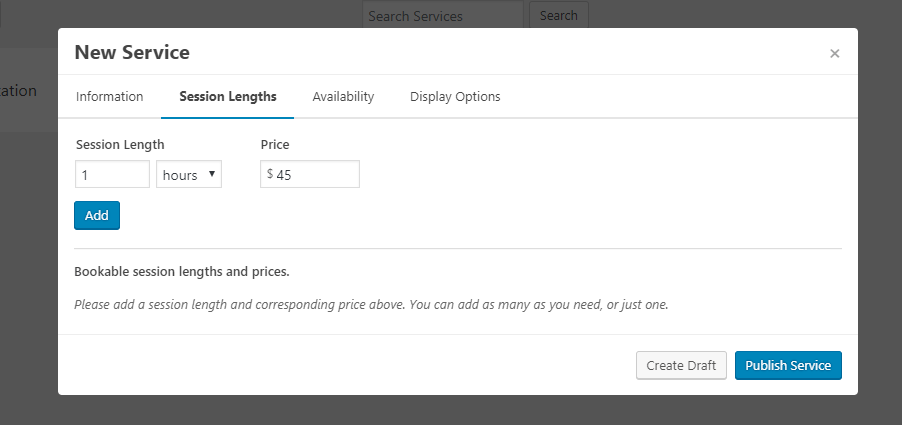In this image, we see a pop-up window titled "New Service" located at the top left in bold black text. Below the title, there are several categories listed: "Information," "Session Lengths," "Availability," and "Display Options." The current focus is on "Session Lengths," which is highlighted in black with the other categories in lighter gray text. A horizontal line underlines "Session Lengths" to indicate selection.

In the main section, the pop-up allows users to specify session details, set to one hour with a price of $45. Below this, a blue button labeled "Add" is prominently displayed. The area captioned "Bookable Session Lengths and Prices" instructs users to add session lengths and corresponding prices, with the flexibility to add multiple options or stick with just one.

At the bottom right corner of the pop-up, there are two action buttons. On the left, a light gray button labeled "Create Draft," and on the right, a blue button with "Publish Service" in white text. The top right corner of the pop-up features a small "X" for closing the window.

The background surrounding the pop-up is a semi-transparent gray, giving a glimpse of the underlying interface. The pop-up itself stands out with a clean white background, ensuring clarity of the information presented.